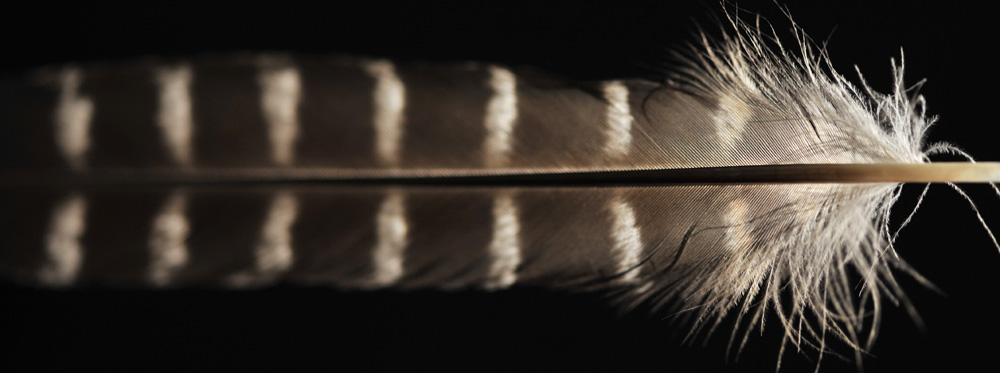This striking photograph is a close-up, macro shot of a single bird's feather set against a completely black background, emphasizing its intricate details. The feather, lying horizontally with the more pointed end (where it was attached to the bird) on the right and the rounded tip on the left, features a dark brown pin needle stem that transitions to white at its base. The right-hand side of the image is in sharp focus, revealing soft, wispy fibers leading to a more rigid structure as you move towards the left. The feather itself is predominantly brown, adorned with white stripes spaced at regular intervals along its length. The composition highlights the delicate, fine strands emanating from the central stem, capturing the symmetrical patterning and textural contrast between the softer and firmer sections. The pure black background ensures that the feather remains the focal point, showcasing the photographer's intent to capture its natural beauty and complexity in exquisite detail.